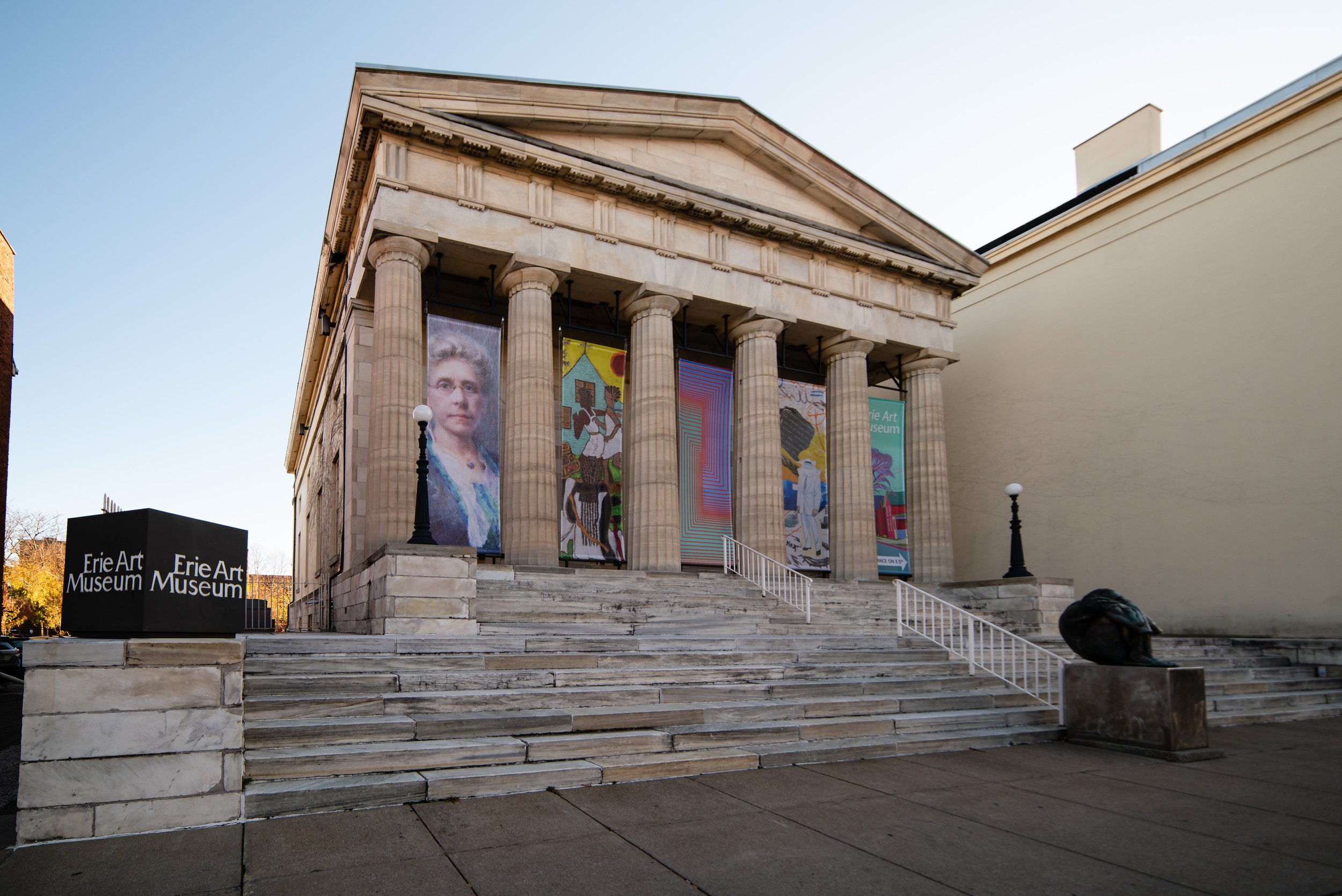The image depicts the Erie Art Museum, prominently featured with a weathered sign on a large, dark cube-shaped post to the left of a grand staircase. The staircase, flanked by stone steps and white railings at its center, leads up to an imposing building supported by six massive pillars at the front. On either side at the top of the steps, there are lamp posts. In front of the building, there are five distinct sections of artwork displayed, with the visible pieces depicting various individuals, including a woman with blonde hair and thin glasses in a blue and white dress, and another featuring a figure in a white outfit with a graffiti-like letter 'Z'. The building is constructed of cement and appears monumental yet modest in scale. The sun’s bright rays cast a glowing effect from the right side against a clear blue sky, further enhancing the majestic ambiance of this outdoor scene. A small concrete landing precedes the ascent of the stairs, adding to the building’s grandeur and sense of welcoming.